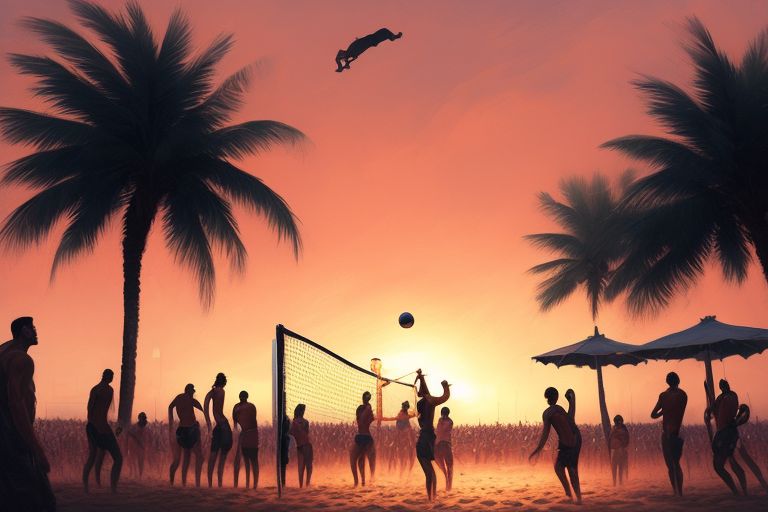A vivid painting depicts a lively beach volleyball scene at sunset, with the sky awash in glowing shades of pink, orange, and yellow. Silhouetted players from two teams vie over the net, with the volleyball suspended mid-air in a dramatic moment, likely a high-stakes spike. In the left foreground, a muscular figure stands out prominently, while on the bottom right, two blue beach umbrellas provide shade for onlookers. The sandy beach appears illuminated, with the kicked-up sand under the players' feet adding a dynamic touch. Palm trees frame the scene—two on the right and a larger one on the left—while throngs of people, possibly waves, fill the background. Intriguingly, a mysterious figure or object hovers high in the sky, capturing the attention of both players and viewers, its nature unclear yet adding a surreal element to the vibrant sunset beach tableau.